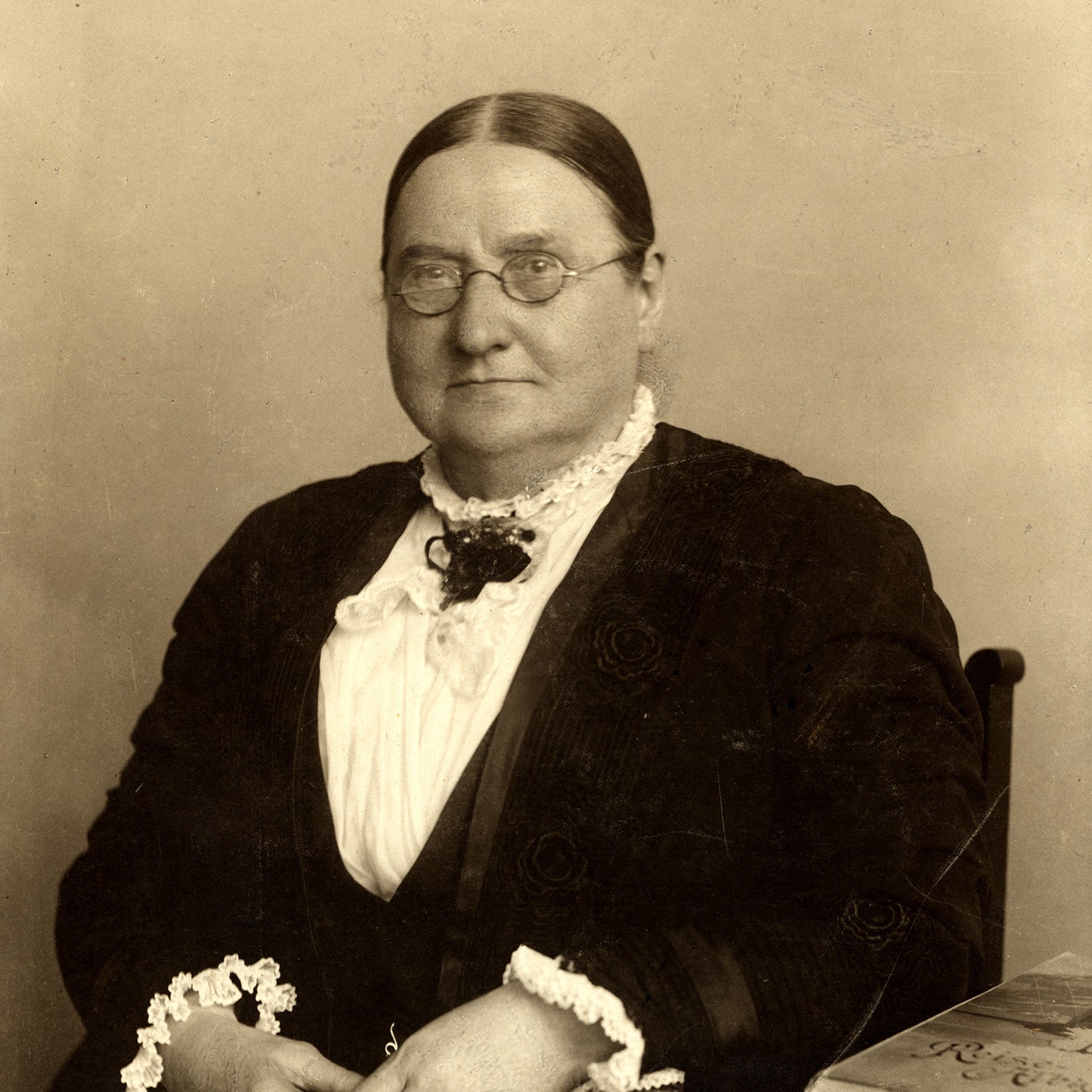A monochrome, sepia-toned photograph captures a woman in her 40s or 50s, of white ethnicity and overweight, seated in a wooden chair against a gray backdrop. She is dressed in formal attire, consisting of a black jacket adorned with a rose print, a white ruffled shirt with frilled collars and sleeves, and a small black bow tie. Her hair is neatly styled with powdered sides, and she wears wire-rimmed, tiny spectacle-style glasses. The woman, identified as Lucy Walker, the second president of the Ladies Alpine Club, gazes directly at the camera. Her hands rest in her lap towards the bottom left of the image, and to the bottom right is a partially visible book with text that appears to read "R.E.I.S.E." This photograph likely commemorates her role in the Ladies Alpine Club.